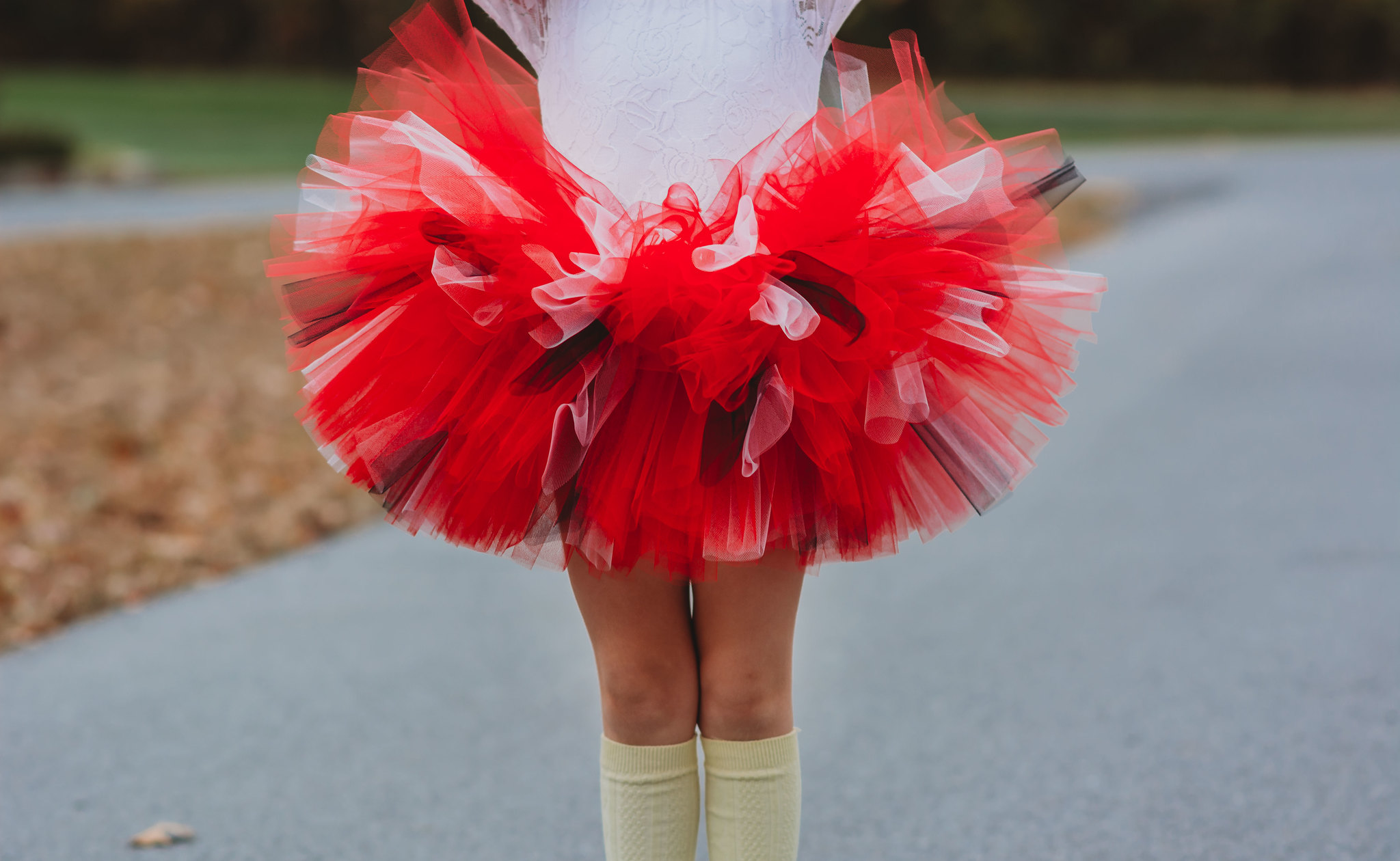In this photograph, a little girl stands outside on a paved driveway amidst a scene of dried autumn leaves and patches of yellowed grass. She's adorned in a vibrant, Halloween-themed tutu, a burst of bright orange, white, and black tulle reminiscent of a poofy bath loofah. Her legs are visible, clad in nearly knee-high, cream-colored socks. The image captures her from the chest down, with her white shirt and raised arms cut off from view, placing full emphasis on her colorful, frilly skirt that extends from her waist to mid-thighs. This playful scene is framed by a median beside the driveway, speckled with dried fall leaves, adding a seasonal touch to the composition.